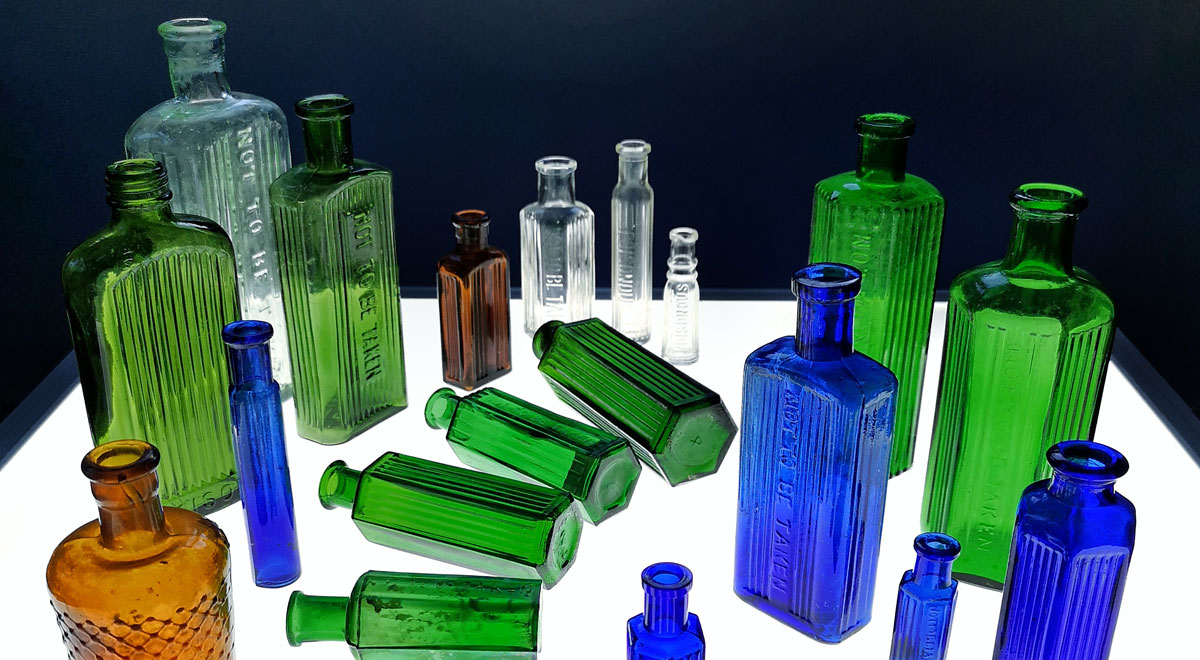The photographic image depicts a collection of 21 glass bottles arranged on a lighted white table in an indoor setting. The collection features various colors and sizes, including blue, green, and clear bottles, as well as a couple of brown ones with copper tones.

Starting from the top right corner, a narrow-necked clear bottle is inscribed with "not to be taken." Adjacent to it are two green bottles: one shaped like a whiskey flask with ridges, and a thinner flask also marked with "not to be taken." Nearby is a small, rectangular brown bottle with a short neck and just half the height of the whiskey flask. Further along the table, a short-necked clear bottle stands next to another clear bottle resembling a whiskey flask, followed by a small clear bottle with a tapered neck. 

Moving right, another green bottle appears, similar in neck style to the previously mentioned "not to be taken" bottle but more cylindrical in shape. There is a series of green bottles along this table, each featuring the same type of glass and ridges, with one situated in the bottom right-hand corner.

Displayed in the bottom corner are four blue bottles: one narrow and rectangular with a short neck, two small ones approximately four inches high with short necks, and another ribbed bottle marked "not to be taken." Lying on the table are four green hexagon-shaped bottles with short necks.

On the bottom left, there is a cylindrical brown and amber-colored bottle with a short neck, and a blue whiskey flask-type bottle. The image includes additional large green brass bottles towards the back left and middle left of the table, as well as three large white bottles in the back row. Overall, the visually striking arrangement of glass bottles, varying in size, color, and design, creates a rich, detailed composition.